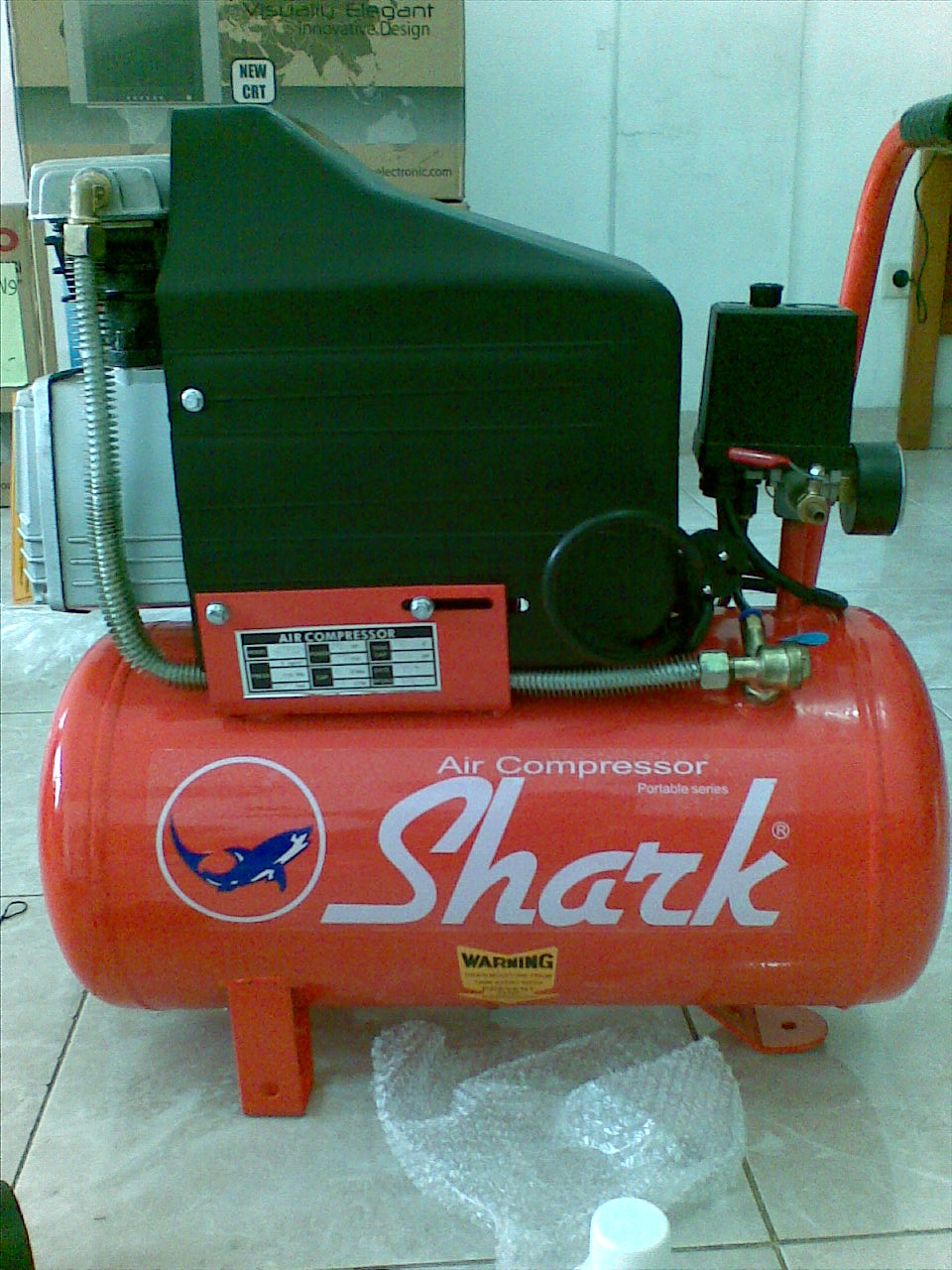This vertically aligned rectangular photograph depicts a red, cylindrical Shark brand air compressor situated in what appears to be a garage. The compressor, which dominates the scene from left to right, is prominently marked with the word "SHARK" in large white letters, with "air compressor" written above in smaller white text. A white circle containing a blue shark logo is visible to the left of the text. The unit rests on two legs and sits on large white stone tiles with gray grout, accompanied by a piece of bubble wrap beneath it. There is a yellow warning label and gauges on the compressor, indicating it might be part of a portable series. The compressor's gray hose extends across the room, connecting to another machine. To the left side, light streaming in suggests the setting is likely a garage. The backdrop features a mix of white wall siding on the right and a creamish sign on the left, adding to the detailed context of the setting.